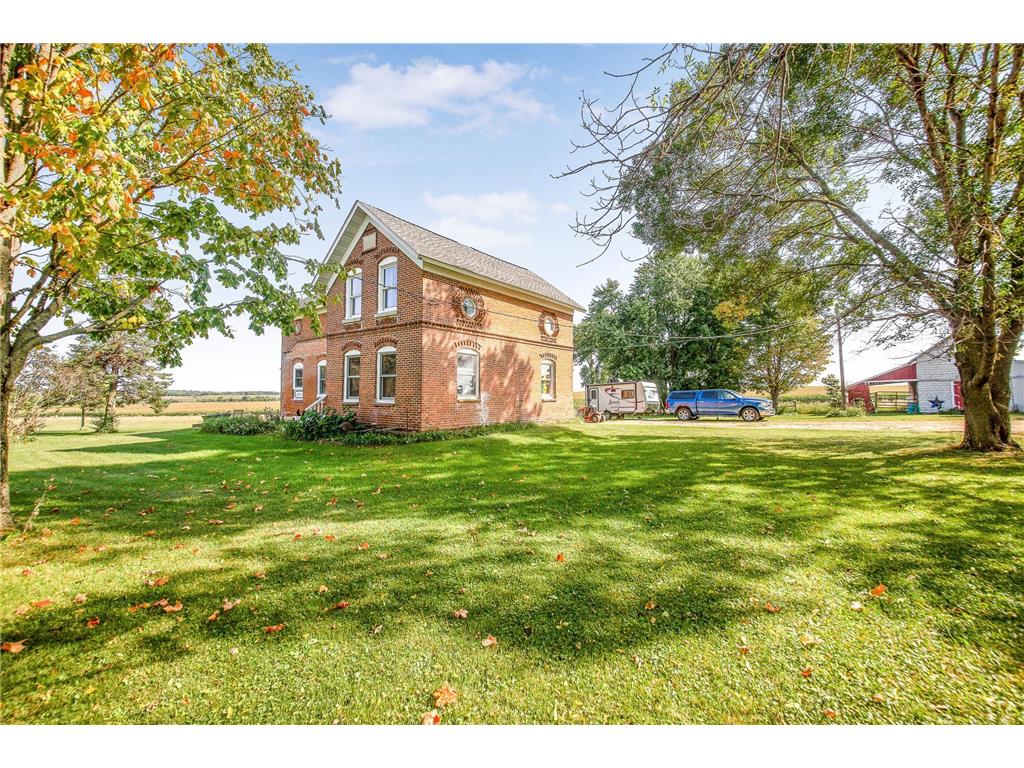This photograph depicts an idyllic country setting featuring a classic red brick farmhouse situated in a lush green field adorned with patches of green and orange fall foliage. The farmhouse, with its grey-tiled roof, has a symmetrical facade with four windows visible on one side and six on the other. The house is framed by two large trees on either side, their tall branches partially bare and leaves scattered on the ground, signaling the transition to autumn. Next to the farmhouse on the right is a blue pickup truck towing a small camper, parked in the driveway. The scene continues with a visually striking barn; primarily red with white accents and a prominent big blue star at its center. A red awning extends from the left side of the barn, through which the entrance to a pasture with fencing is faintly visible. The background features additional trees near the barn, all beneath a mostly clear blue sky dotted with a few fluffy clouds, brightly illuminated by the sun. This picturesque snapshot captures the essence of rural tranquility.